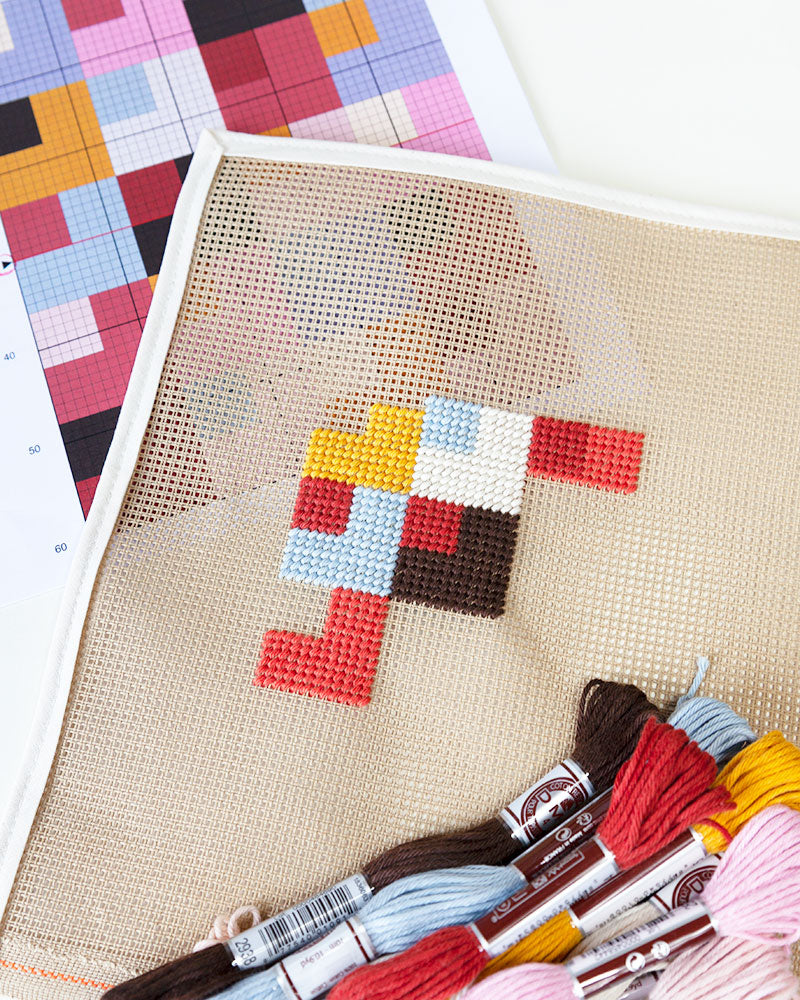The image showcases a detailed embroidery or cross-stitch project set up on a white surface, possibly for a professional photograph. It prominently features a piece of paper in the top left, bearing a grid pattern with various colored boxes—red, orange, blue, white, and black. Overlaying this paper, in the bottom right, is a beige mesh cloth with a white trim that has small holes designed for sewing through. The mesh displays a partially completed pattern that mirrors the design on the paper, with colors including red, brown, white, blue, and yellow. Bundles of embroidery thread in pink, red, yellow, light blue, brown, mustard, black, and maroon, some still in their original wrapping, are laid out on top of the mesh. The project appears to be about one-third finished, with the intricate squares within squares pattern gradually taking shape, hinting at a quilt-like final design. Small, indistinct labels can be seen on the threads, adding to the meticulous setup of this crafting endeavor.